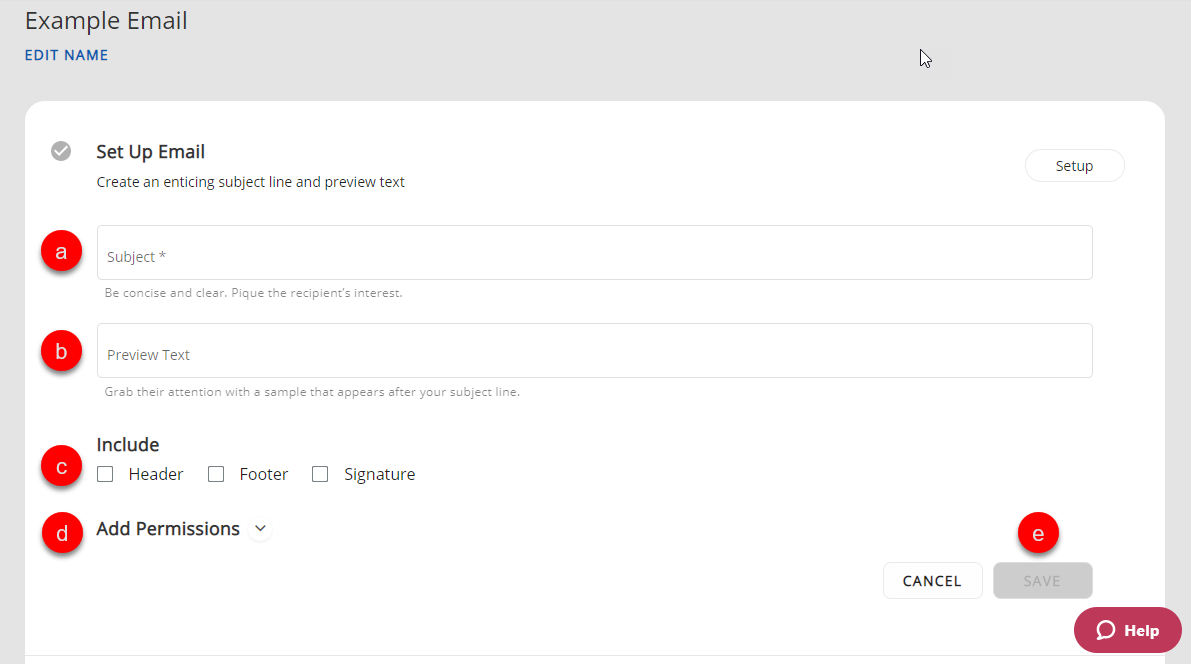The image depicts a snapshot of a website providing an example of how to send an email. In the top left corner, the page is titled "Example Email." The main section of the snapshot contains two fields: one for inputting the email subject and another for preview text, labeled A and B respectively. 

Additionally, there are three other sections labeled C, D, and E:
- Section C displays three unchecked checkboxes labeled "Header," "Footer," and "Signature."
- Section D includes the text "Add Permissions."
- Section E, situated in the bottom right corner, offers options to "Save" and "Cancel" with two side-by-side buttons. This section also features a "Help" button, which is oval-shaped and dark red, almost burgundy, with the word "Help" on it.

Overall, this snapshot illustrates how to set up an email, preview its text, and input the subject.